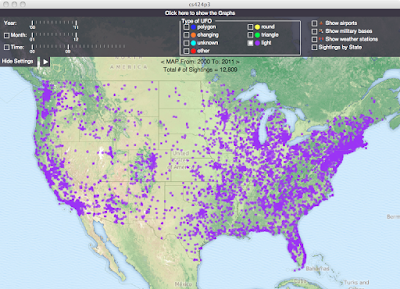This image features a detailed map labeled "Click Lyons to show the type of LFO," showcasing various data points and color-coded keys. At the top of the map, the title "North America" is visible, indicating the geographical focus. It also notes "Map from 2000 to 2011" and mentions a "Total of sightings: 12,800" on the right side.

The map is rich in visual information, with colored dots indicating different types of Low-Frequency Oscillations (LFO). The legend categorizes these as follows:
- Polygon: Blue
- Sound: Yellow
- Triangle: Green
- Light: Purple
- Unknown: Light Blue
- Either: Red

The map itself displays green areas representing vegetation and brown areas denoting land. A notable feature is the prevalence of purple dots, signifying a high number of light-related LFO sightings. Additionally, the letters "C" appear in both the bottom right and bottom left corners, potentially indicating cardinal directions or map legends.

The top section of the image, containing some of the text, is slightly blurry, but the overall information remains comprehensible. Purple, or light-related LFOs, dominate the data points, making them a significant focus of this visual representation.